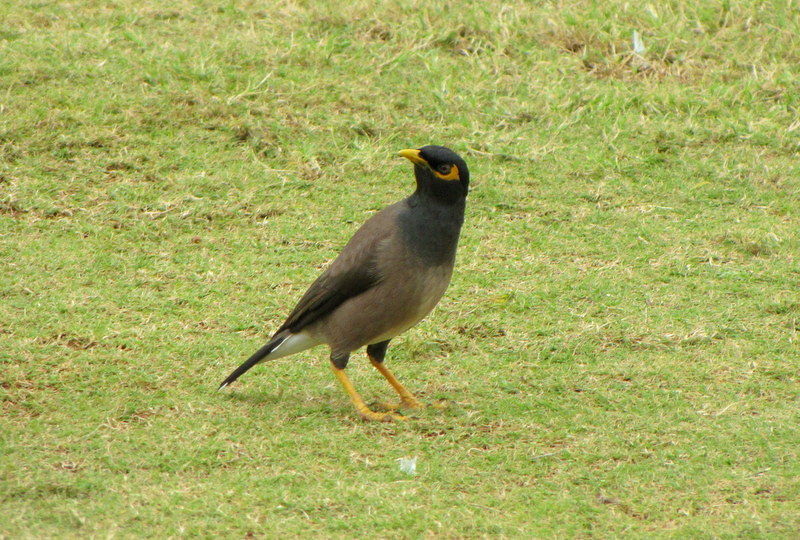A bird stands prominently in the center of a mostly flat, grass-covered field. The field is a mix of short light green and brown grass, with some hay-like patches and spots of visible dirt. There is a small white piece of trash on the ground in front of the bird.

The bird has a striking appearance featuring a blend of colors. Its head is a deep black, and its body transitions from dark gray near the neck to a lighter brown and gray as you move downward. The tail and wings have black tips, with the front top side of the tail also being black. Underneath the tail, the bird is completely white. The bird's bright yellow beak extends into a small bright yellow patch around its black eye, making the eye stand out. It also has long, bright yellow legs that match its beak.

The bird is about the height of a crow, and it exudes an almost unique combination of traits reminiscent of a crow and a penguin. It faces toward the right side of the image with its body but has its head turned to the left, gazing slightly away from the camera.